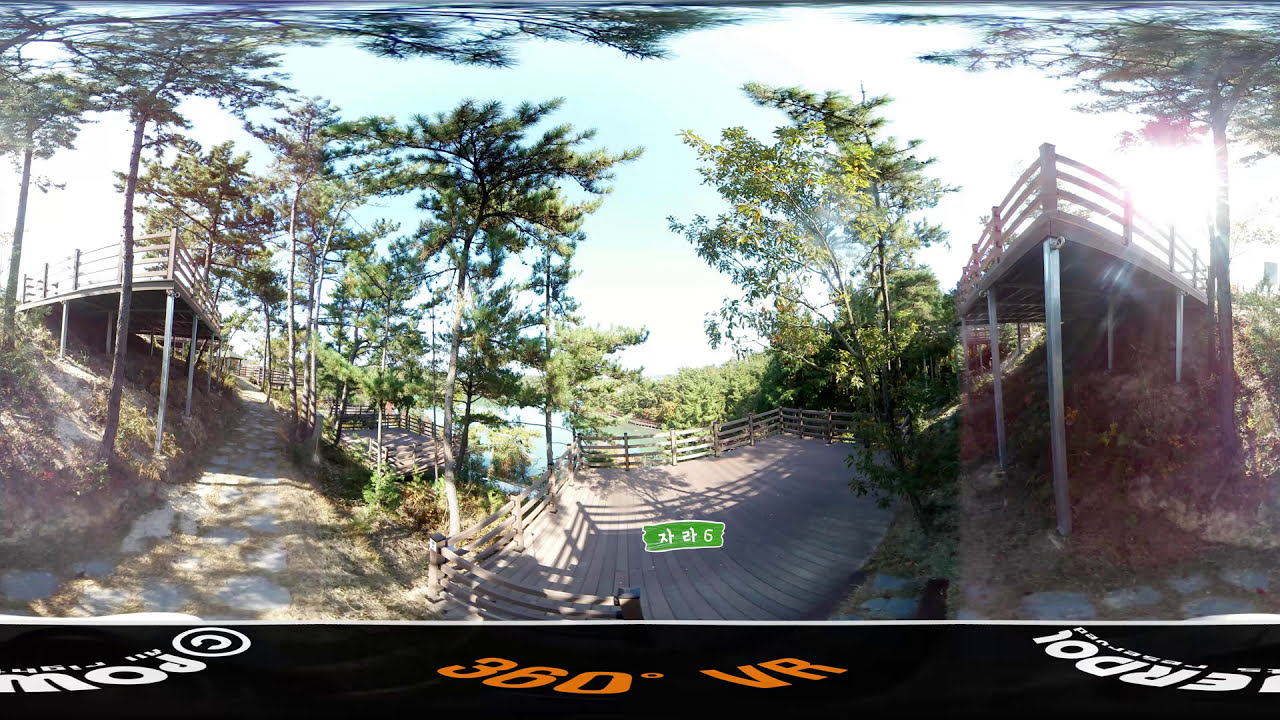The image is a 360-degree panoramic photograph designed for VR, depicting a scenic landscape with multiple wooden observation decks built over a steep, tree-covered hill. In the center of the image is a large, square wooden deck enclosed by a fence, offering a view of a lake or river in the background. To the left and right of the central deck are additional elevated wooden platforms on stilts, facing each other and overlooking the dirt paths running beneath them. The sky above is bright and sunny, casting light on the dense forest that surrounds the entire scene. A caption at the bottom of the image reads "360 degree VR" in yellow or orange writing against a black band.